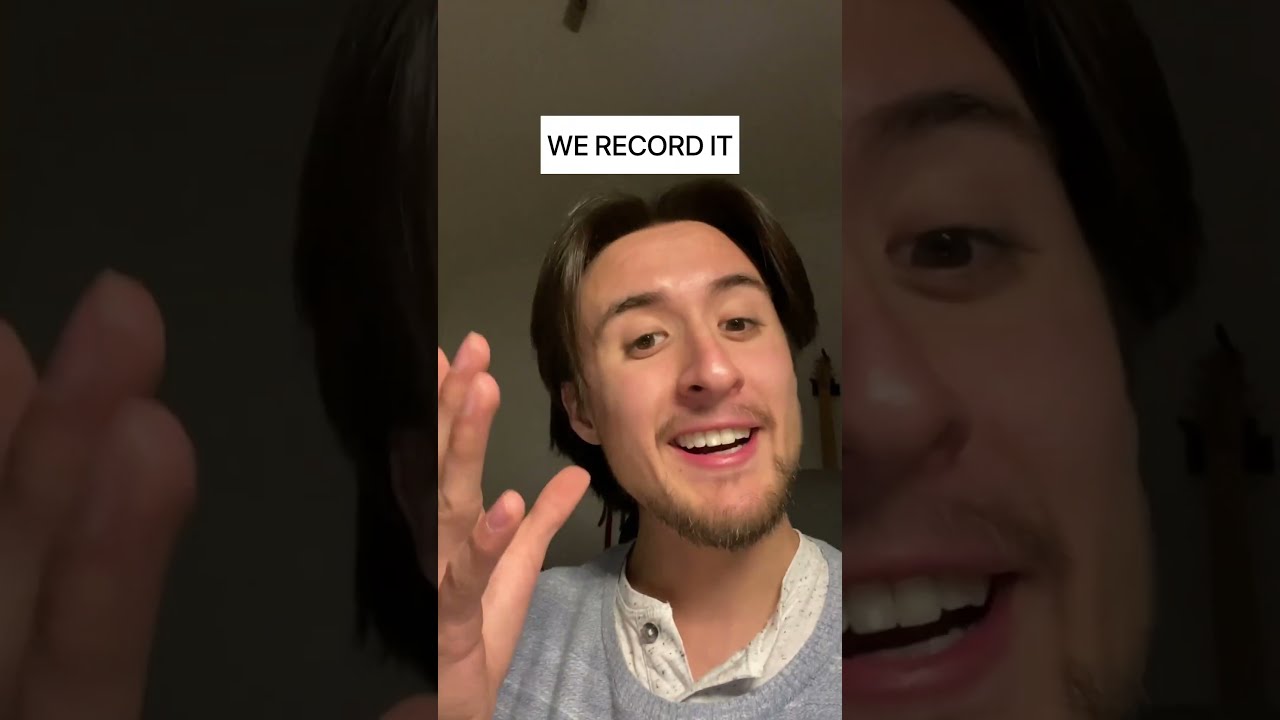The photo, seemingly a still shot from a video call, captures a man with brown hair parted in the middle and reaching down to his ears, complemented by a goatee and mustache. He is gesturing with his right hand up and fingers pointing, while smiling and talking. The man, who appears to be white, is wearing a gray cardigan over a white shirt. The scene suggests he is in a bedroom, evidenced by the portion of a ceiling fan and a guitar hanging on the wall behind him. Above his head, a white bar spans horizontally with the caption "we record it" written in black letters. The image is bordered with a repeated blurred version of itself, adding depth to the photo. The dominant colors present are black, white, gray, beige, brown, and red.